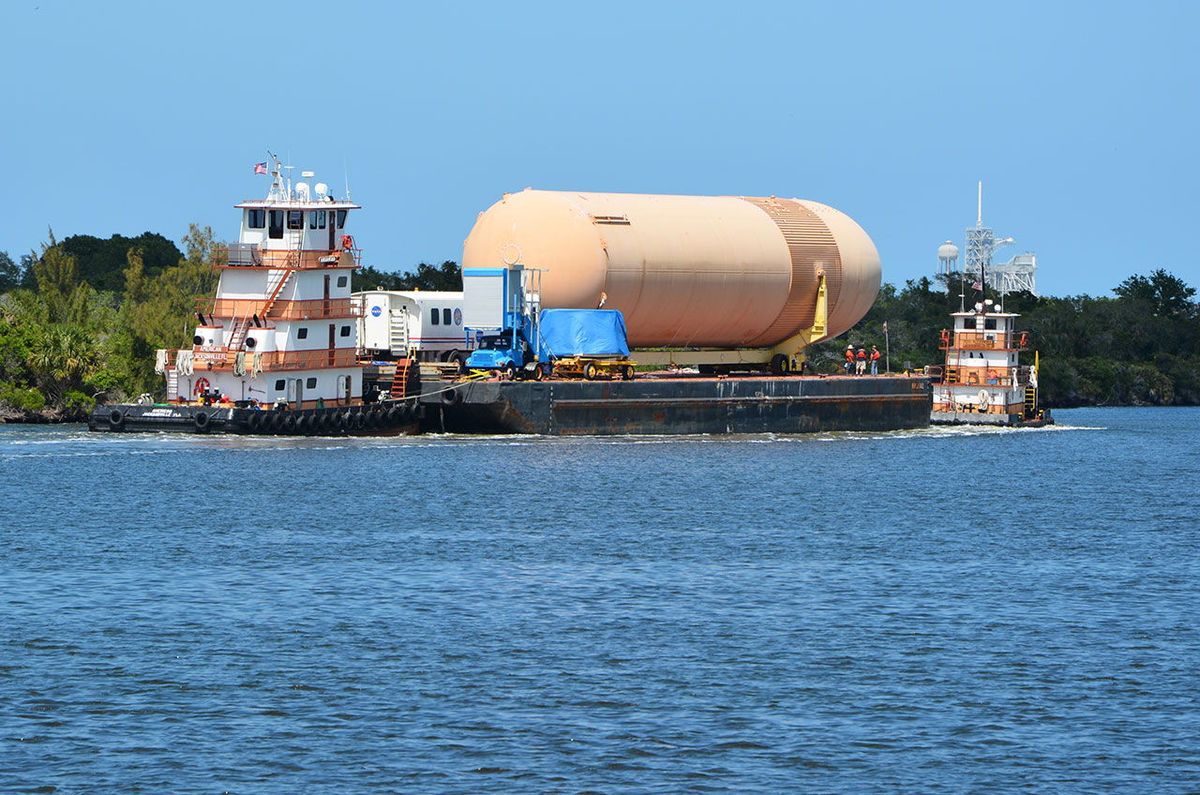The photograph captures a serene, bright blue lake on a clear day with calm waters. Dominating the center of the image is a large, dark gray-black barge. It has a flat structure with a four-tiered white superstructure featuring stairs at the front and a substantial, cylindrical, tan-colored tank near the back. This tank is large and round, resembling a fuel container, and there are three tiny people standing beneath it on the barge. The barge appears to be flanked by two tugboats, one in front and one to the right rear, suggesting that these tugboats are maneuvering the barge. The image also includes a lush, green landmass stretching from the left to the right of the photo, partially obscured by the barge. The sky is a vivid blue, contributing to the overall tranquil and bright atmosphere of the scene.